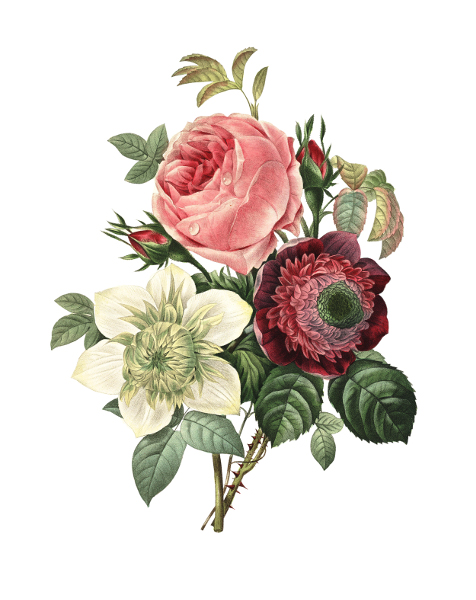The image depicts a detailed and sophisticated floral arrangement against a neutral white background. At the top of the arrangement is a pink rose, accompanied by smaller, yet-to-bloom rose buds on a thick, thorn-covered green stem. Below the rose, on the left, is a six-petaled white flower with a prominent green and yellow bulbous center, attached to a smooth green stem adorned with small, teardrop-shaped leaves. To the right, there is a striking large flower with outer petals in a dark red hue and inner petals in a lighter pink, encircling a green center. This flower is connected to a smooth stem with rounder, darker green leaves. The composition includes a diverse palette of colors ranging from pinks to reds, off-whites, and various shades of green, with some leaves showing a transition in color to yellow and pink. The overall clean, fresh, and elegant display highlights both the beauty of the individual flowers and their harmonious arrangement.